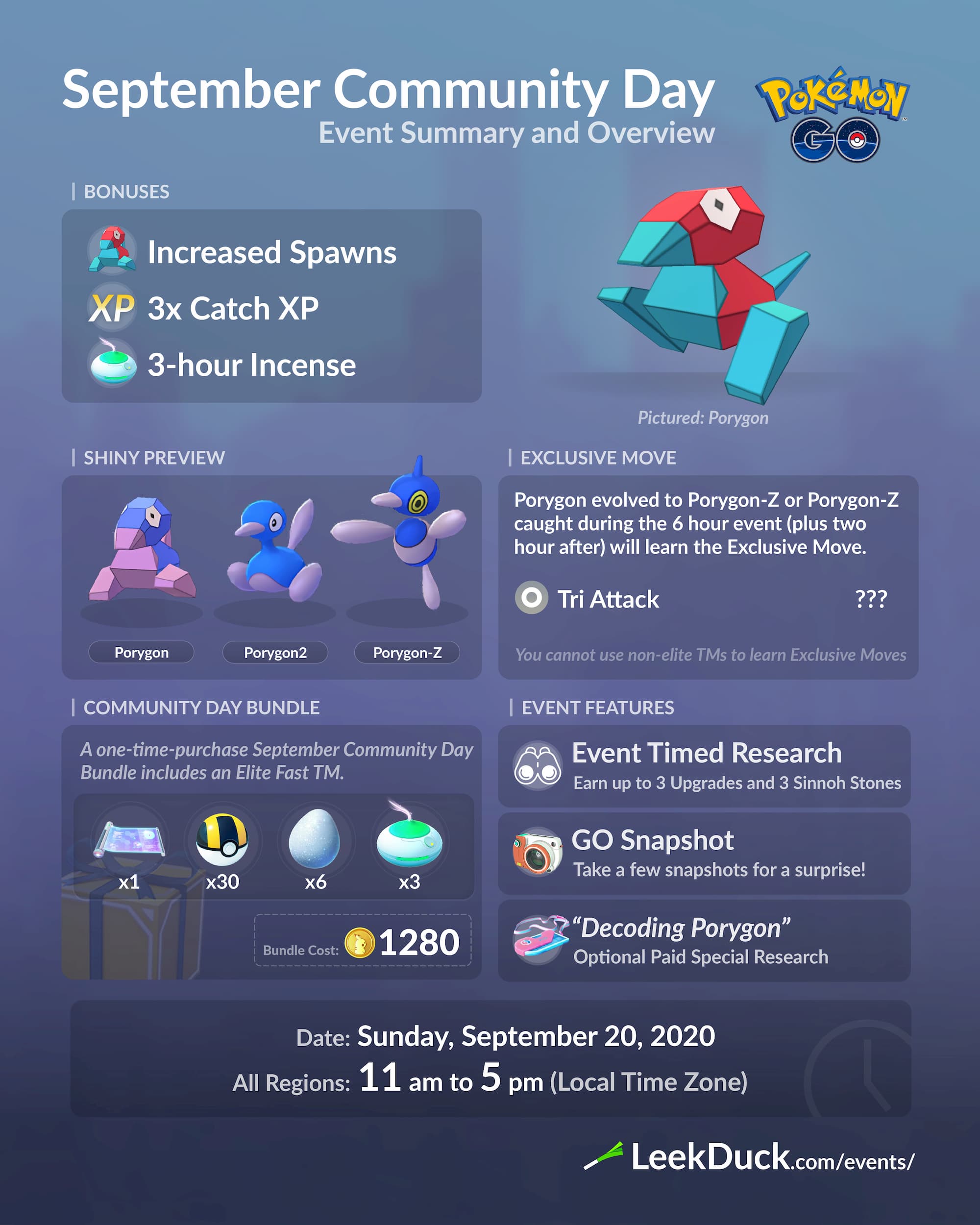**Poster Description for Pokémon GO September Community Day Event**

The vibrant poster is designed with a dark and pale blue gradient background that emphasizes various event details. At the very top right corner, the iconic Pokémon GO logo stands out. To the left of the logo, spanning from the top left to the center, bold, large white text announces "September Community Day." Directly below, in smaller text, it says "Event Summary and Overview."

The poster features an eye-catching image of Porygon, a distinctive blue and red low-poly Pokémon with a visible eye, positioned to the right. Adjacent to this image, on the left, is a translucent dark box containing a detailed list of event features complemented by corresponding images:

1. **Increased Spawns** - Represented by another image of Porygon.
2. **3x Catch XP** - Accompanied by white text "XP."
3. **3-Hour Incense** - Illustrated with an image of a green and white circle.

Beneath this list are four different segments providing comprehensive information about the Porygon Community Day and associated event features, such as:
- Bundles
- Exclusive Moves
- Event Timed Research
- The evolution of shiny Porygon
- Ghost Snapshot

At the bottom center of the poster, within an opaque box, there's a date and time section marked by a clock symbol. It reads "Sunday, September 20, 2020," followed by "All Regions, 11am to 5pm local time zone." Finally, the bottom right corner features a picture of a leak with accompanying white text noting "LeakDuck.com/events."

This detailed and visually engaging poster provides a comprehensive overview of the exciting Pokémon GO September Community Day event, ensuring players are well-informed about all features and timings.